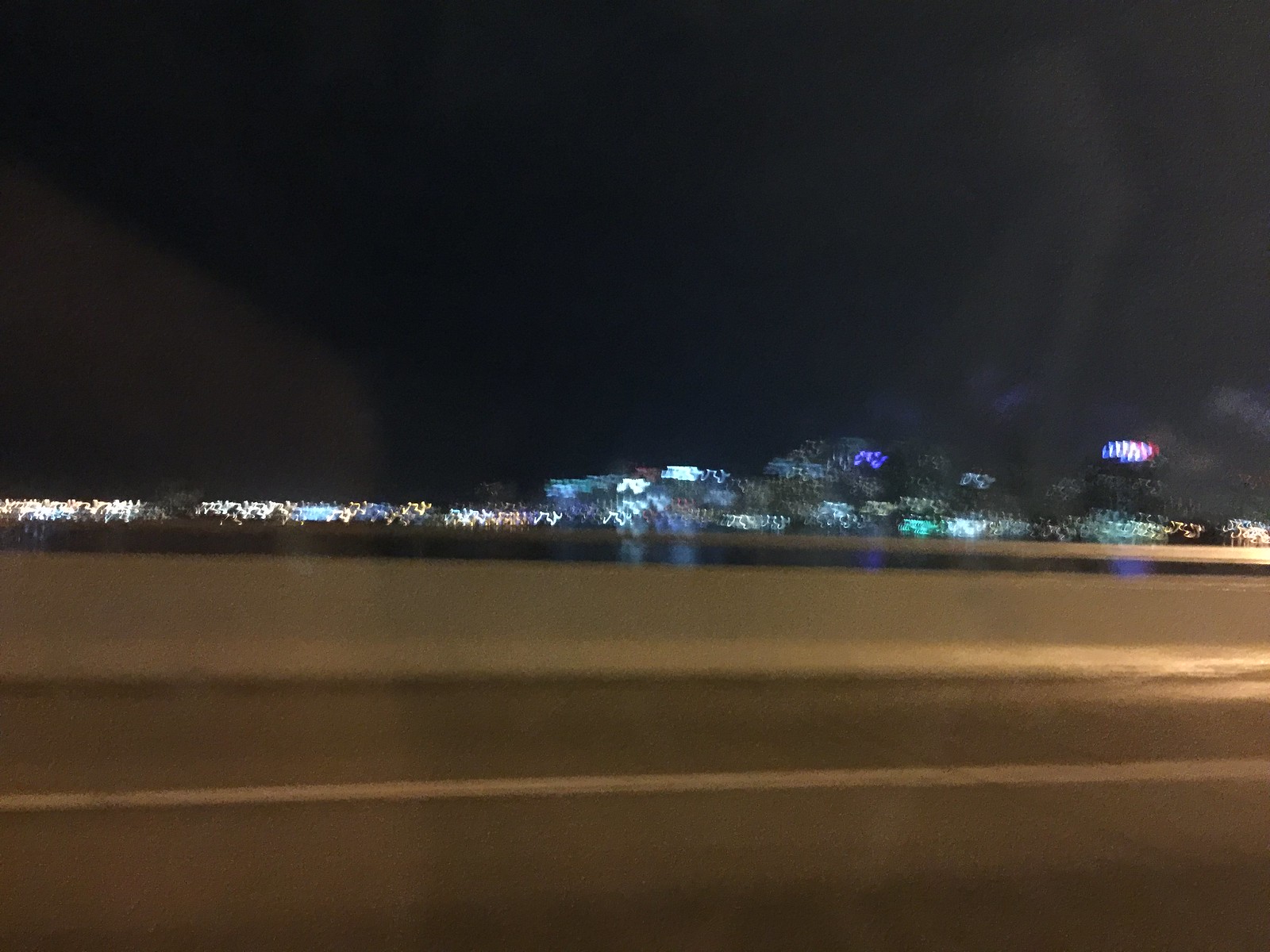This abstract evening photograph captures a blurred, metropolitan scene centered around an expansive highway. Dominating the foreground, a concrete guardrail delineates the road, leading the viewer's eye toward the distant cityscape. The buildings in the background appear softened and indistinct due to the motion blur, resulting in an ethereal glow of diffused lights. The sky above is a deep, midnight black, interrupted by wisps of what could be clouds or smoke, adding a moody, atmospheric layer to the composition. The whole image exudes a sense of urban serenity, filtered through the lens of twilight and motion.